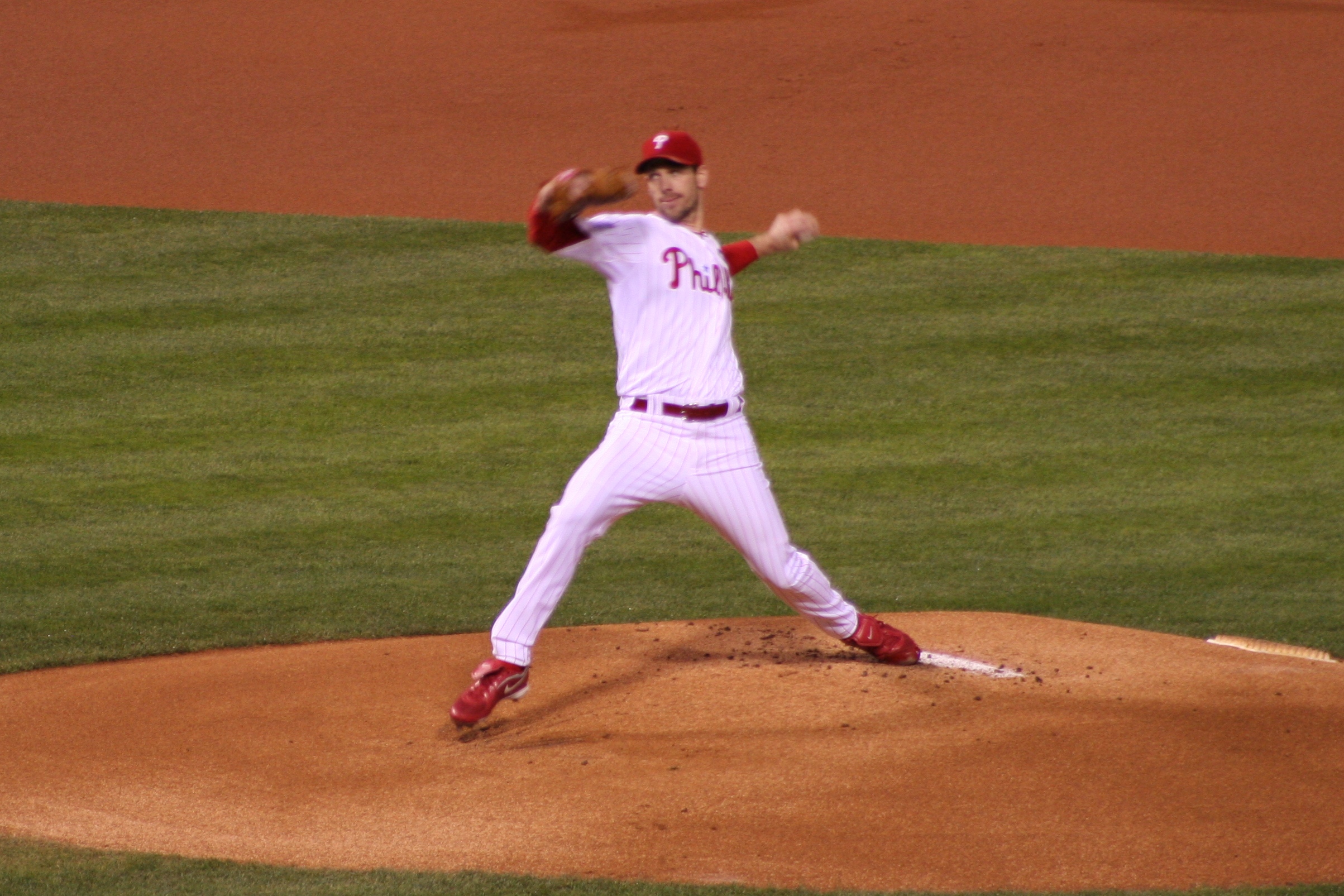In this slightly blurry image, a Philadelphia Phillies baseball player is captured mid-pitch on the mound, ready to throw the ball. He is wearing the iconic Phillies uniform: a white jersey and pants adorned with vertical red pinstripes, and "Phillies" written in red across the chest. Underneath his jersey, he sports a red, three-quarter sleeve shirt, and a red belt cinches his uniform. His red Nike cleats stand firmly on the pitcher's mound, with his left foot resting on the white pitcher's rubber. The player wears a red cap featuring a white "P" and is holding a baseball in his left hand, while his right arm, clad in a brown glove, extends outward in preparation for the pitch. Surrounding him, the well-maintained, short green grass of the infield contrasts with the neatly groomed brown dirt of the baseball field.